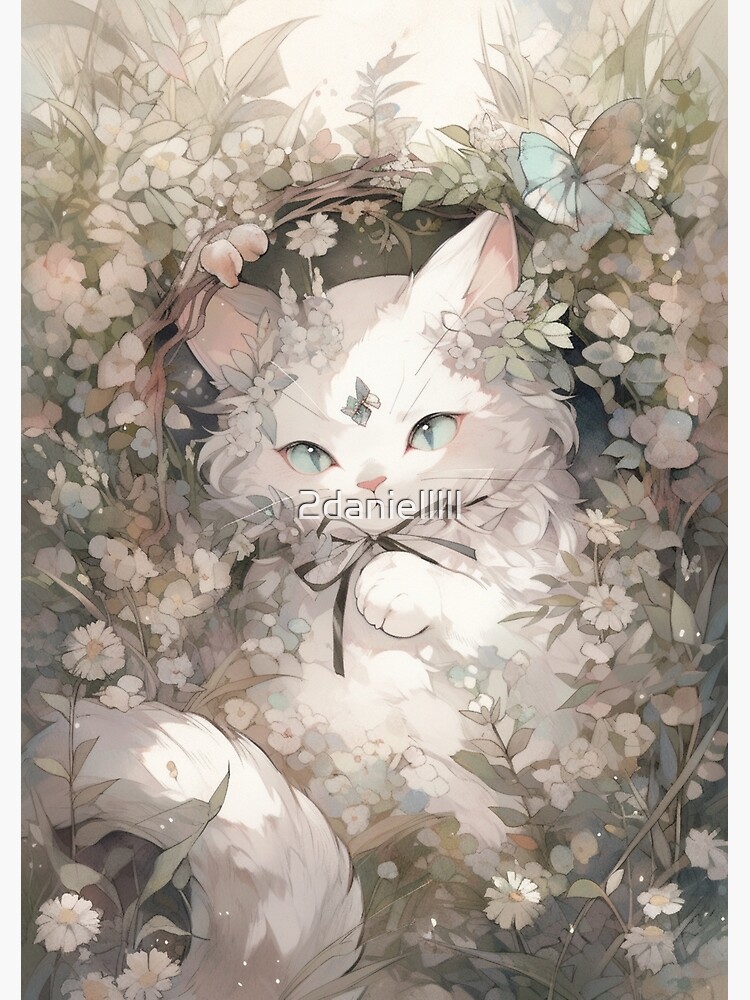This digital illustration depicts a fluffy white kitten with long fur, sitting amidst a vibrant array of pastel flowers and plants. The kitten, which is facing the viewer with its blue-green eyes, has a gray and white bow tied around its neck. A leaf gently rests between the kitten’s ears, and a butterfly hovers just above its head, adding a whimsical touch.

The background boasts a soft gray tone, complementing the delicate colors of blue, red, green, and pastel hues found throughout the flowers and foliage. The kitten's fluffy tail curls up to the left side of the image, and its long fur radiates a soft, plush texture. Subtle white flowers with yellow centers, along with light green and white leaves, create a serene and gentle atmosphere around the kitten.

The bottom right corner of the image contains a watermark that reads “to Danielle” in a subtle, small font. The overall artwork blends light and shade seamlessly, with slightly darker tones in the bottom corners, enhancing the dreamy quality. The kitten’s charming expression and the enchanting floral setting make this image an adorable and serene depiction.